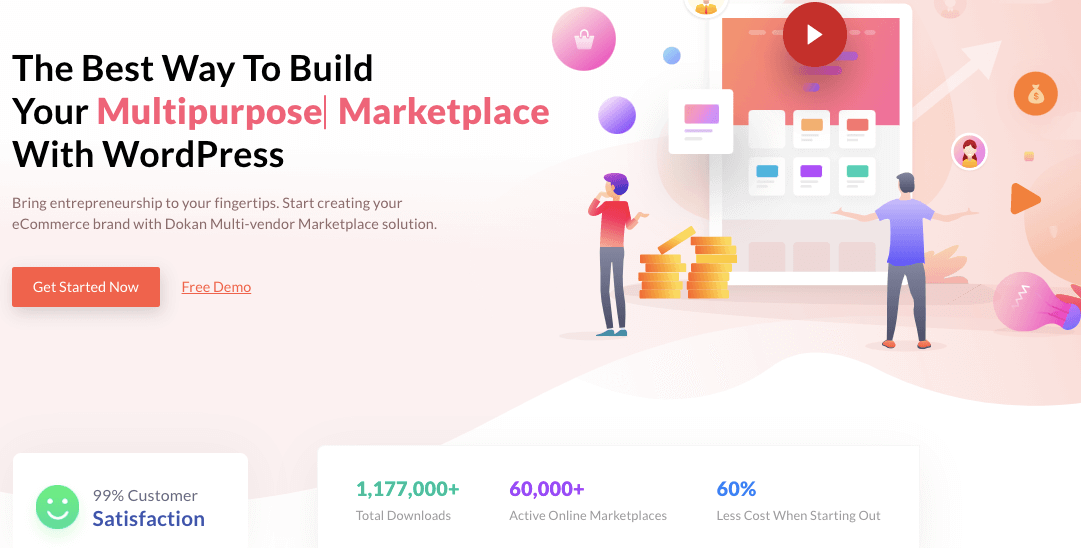Here is a cleaned-up and detailed descriptive caption for the image:

---

This screenshot features a website promoting its WordPress platform for building multi-purpose marketplaces. Dominating the center of the image is bold text stating, "The best way to build your multi-purpose marketplace with WordPress." Surrounding this are vibrant graphics, including coins symbolizing financial transactions, a person standing with arms outspread conveying empowerment, and a woman seemingly contemplating her choices. Additional elements include a play button, an arrow, and a light bulb, all representing dynamic features and innovative ideas.

Towards the bottom, a prominent call-to-action button reading "Get Started Now" stands out with a pinkish hue, urging users to explore further. It promotes the availability of a free demo. Highlighted statistics are also present: "99% customer satisfaction" is marked in blue text alongside a smiling face icon in green. "1,177,000 full downloads" is displayed in a mix of green and purple, emphasizing the platform's wide reach, while "60,000 active online marketplaces" follows suit. Additionally, "60% less cost when starting out" is featured in blue text. The entire site boasts a sleek, gradient effect in its design, adding to its modern and appealing look.